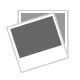The image displays a roughly textured metallic star-like sculpture, potentially made of cast iron, but painted in a bronze, gold, or slightly golden color. The sculpture features a central circular cutout surrounded by spear-like, very pointy triangular rays that fan outwards, resembling a sunburst or a traditional Christmas star. This sculptural piece is set against a plain white background, which appears to be a wall. The photograph only captures the bottom left portion of the star, cutting off the upper part and the right side, leaving the full shape and structure partially obscured. The absence of surrounding text or additional context, combined with the indoor setting, suggests a focus on the artistic details and metallic quality of the sculpture, which evokes imagery commonly associated with Christmas or nativity scenes.